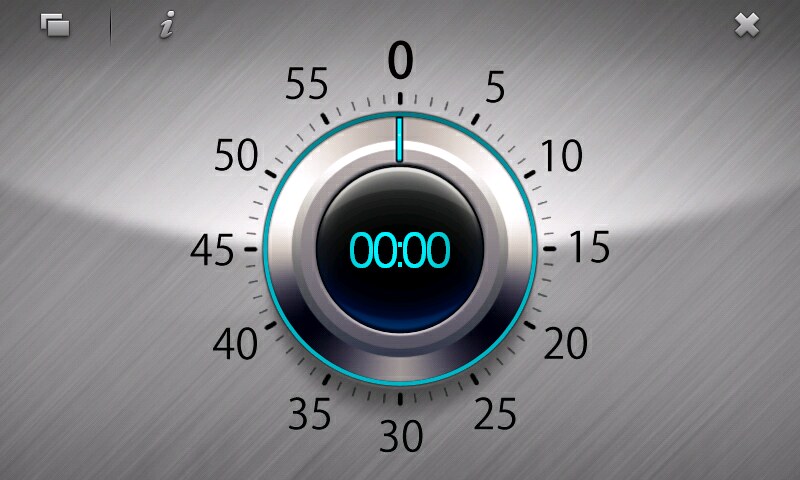The image appears to be a screenshot of a digital interface, likely from a video screen graphic, displaying a modern, high-quality digital timer. The background is a gray, metal-like texture with diagonal streaks, shaded to be lighter on the upper half. In the upper left-hand corner, there are two small icons: a file folder icon and an information (eye) symbol. There is also a white 'X' to close the window in the upper right-hand corner.

Dominating the center of the screen is a speedometer-like dial, intricately designed with a digital, teal blue (aqua) font. The circular dial is bordered in aqua and features black numerals around its perimeter, marked in increments of five: 0, 5, 10, 15, and so forth up to 55. Between these numbers are smaller tick marks for more precise readings. At the very center of the dial is a black circle displaying "00:00" in teal blue, with a needle pointing to zero, indicating that the timer is set to zero. The overall design mimics a traditional physical timer but in a digital, computer-based format.